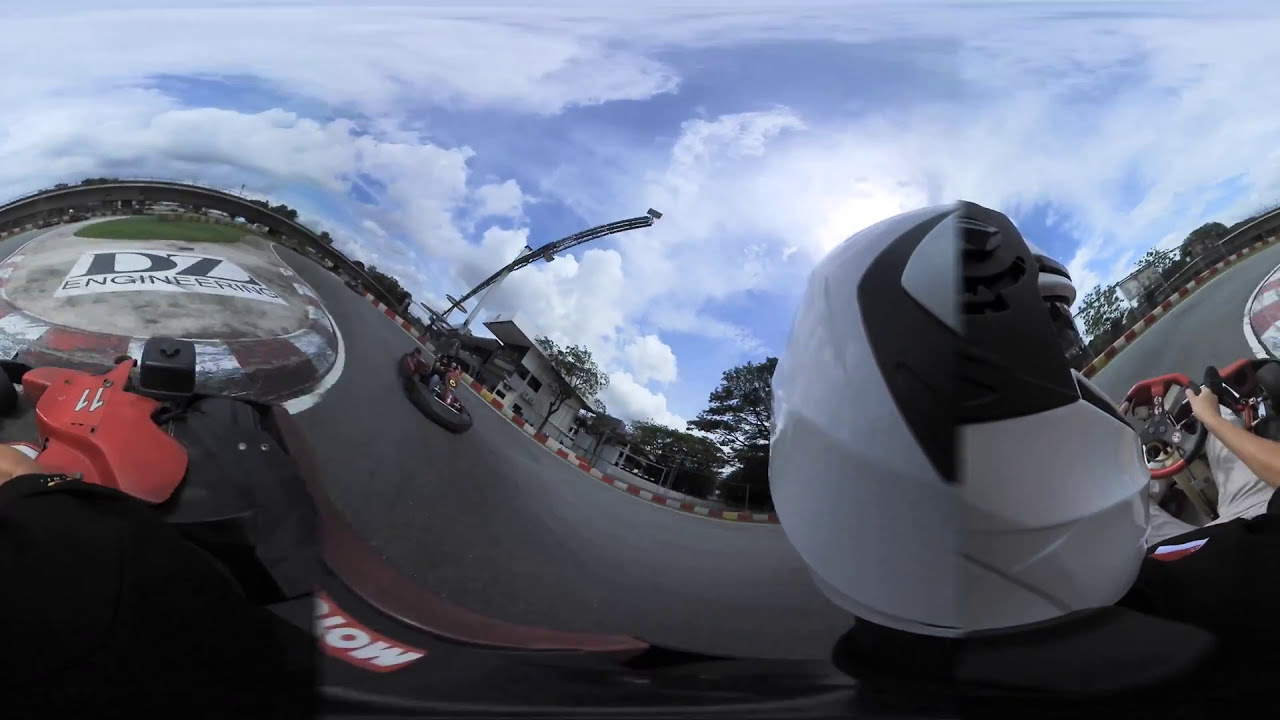This image portrays a go-kart park with a distinctive vertical, rectangular orientation, possibly altered or taken with an unusual camera lens, resulting in a wavy, angled appearance. Dominating the foreground is the view from within a go-kart, showcasing a white-helmeted driver gripping the steering wheel. In the background, a black-bumpered go-kart navigates a dark gray concrete track bordered by alternating red and white curbs. On the left side of the image, a concrete area partially raises off the track, adorned with the text "DZ Engineering" and accompanied by a patch of grass. Surrounding the track, trees and buildings are visible, set against a backdrop of blue sky filled with gray and white clouds, through which sunlight streams.